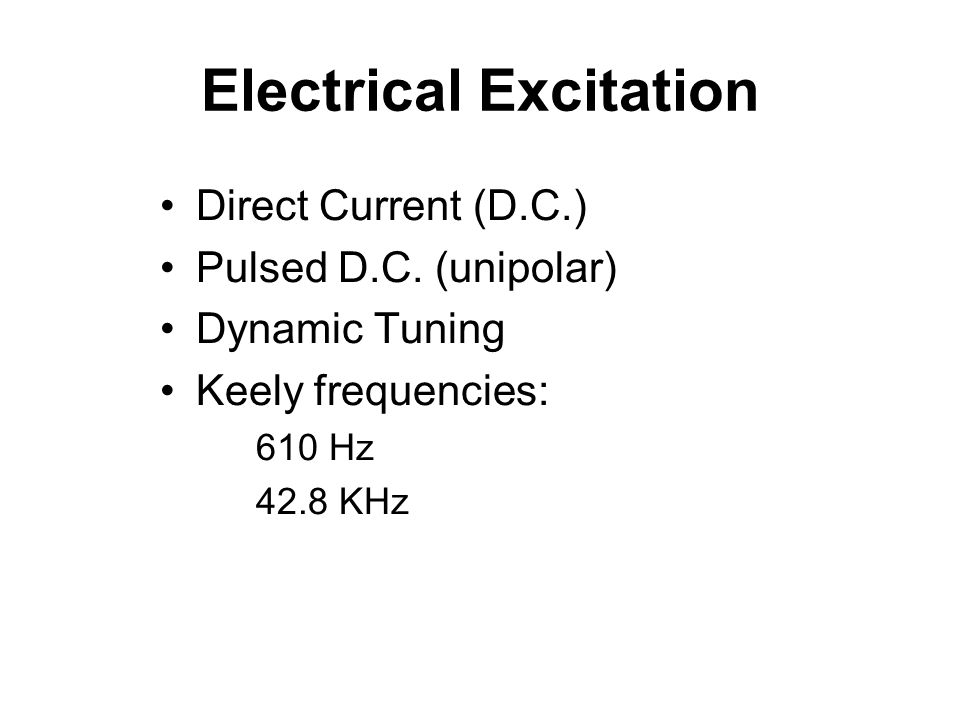The image displays black text on a solid white background, resembling a list on a Microsoft Word document or PowerPoint slide. At the top, in a bolded sans serif font, the title "Electrical Excitation" is prominent. Below the title are four bulleted points. The first bullet states "Direct Current" with "DC" in parentheses. The second reads "Pulsed DC" with "Unipolar" in parentheses. The third bullet point simply says "Dynamic Tuning." The fourth bullet point is labeled "Keely Frequencies:" followed by two indented sub-points: "610 Hertz" and "42.8 kilohertz."